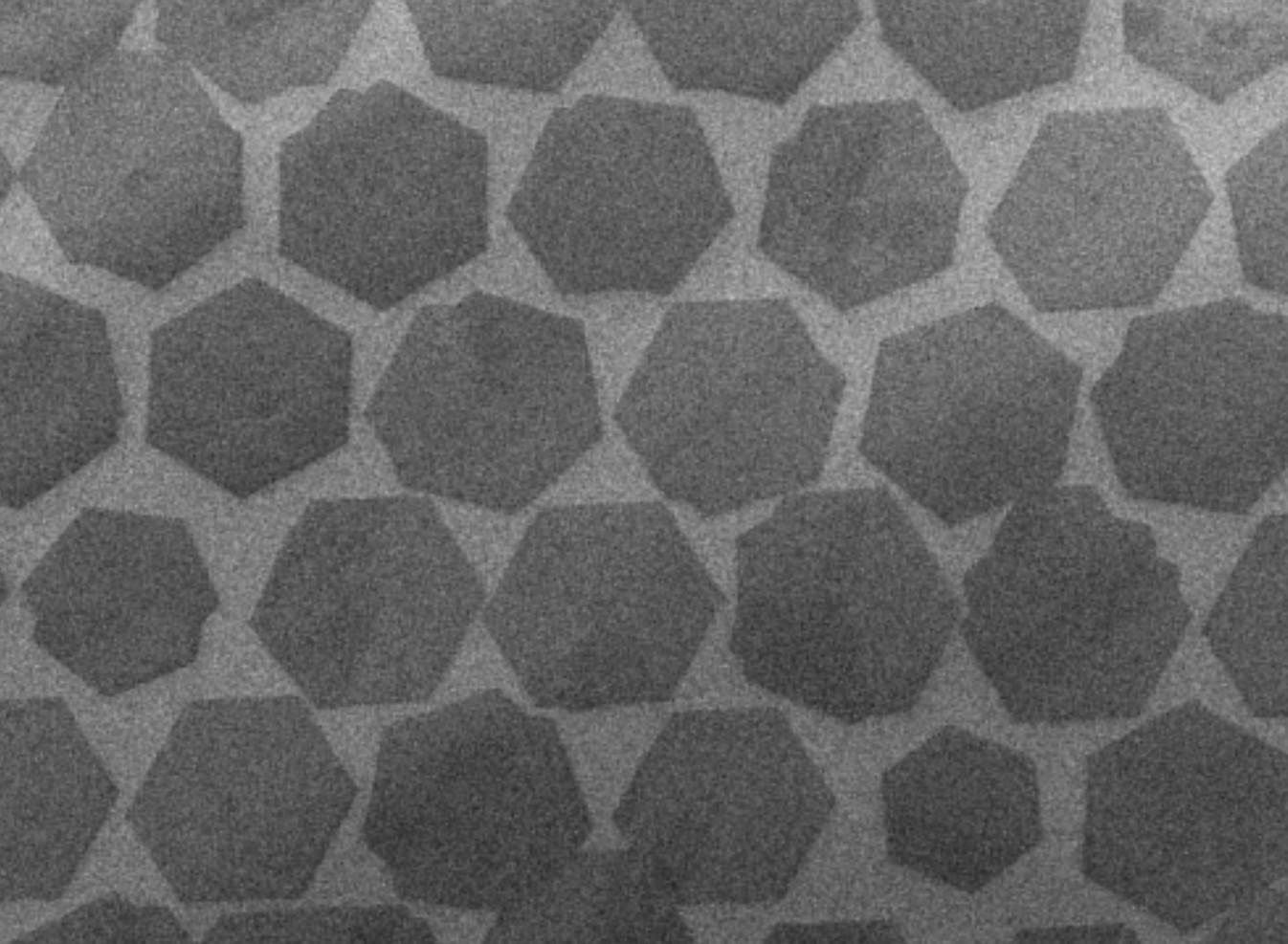This image features a close-up view of a textured surface displaying an abstract pattern composed of various shades of gray. The pattern consists of numerous six-sided figures, predominantly hexagonal, which exhibit a slightly grainy texture and varying degrees of blur. These hexagons, interspersed with a medium gray color, are surrounded by a lighter gray backdrop, creating a striking contrast that contributes to the complexity of the design. The hexagonal shapes, though mostly consistent, also include a few irregular, rounded, or slightly rough-edged figures. There's also one distinct shape with a more squared side and a ruffled top area, setting it apart from the rest. The entire image suggests the detailed texture of a fabric, surface of stone, or possibly an abstract, close-up black and white photograph, highlighting the intricate interplay of fibers or grains throughout the composition.